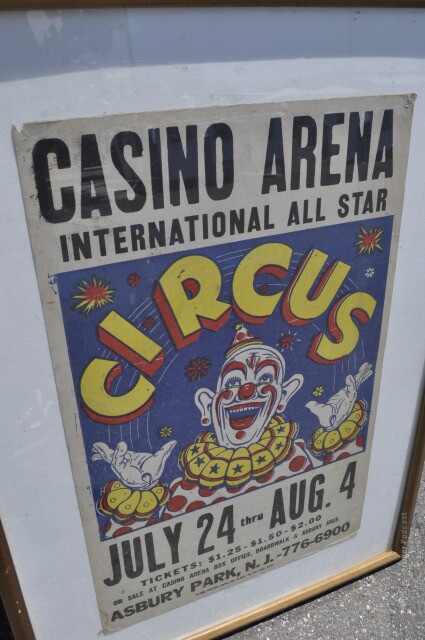In the image, we see a vibrant sign prominently displayed in the center of a paved, gray asphalt road. The outdoor setting, captured in the middle of the day, features the sign which appears to be protected behind glass. The sign is a paper poster mounted on what looks like a white board, presenting a mix of colors including light blue, white, black, gray, off-white, yellow, red, black, and tan. It announces the "Casino Arena International All-Star Circus," held from July 24th through August 4th in Asbury Park, New Jersey. The ticket prices listed are $1.25, $1.50, and $2. The top of the sign has bold black letters, while a blue square in the center, with large yellow and red letters, highlights the word "circus." Beneath this, there's an illustrated clown with a mouth open, looking upwards with hands raised, adorned with a yellow collar, red and blue face paint, and a white face. The bottom portion, which includes the event dates, has additional black text that is somewhat hard to discern. The overall scene suggests the sign is positioned outside, possibly near the venue of the event it advertises.